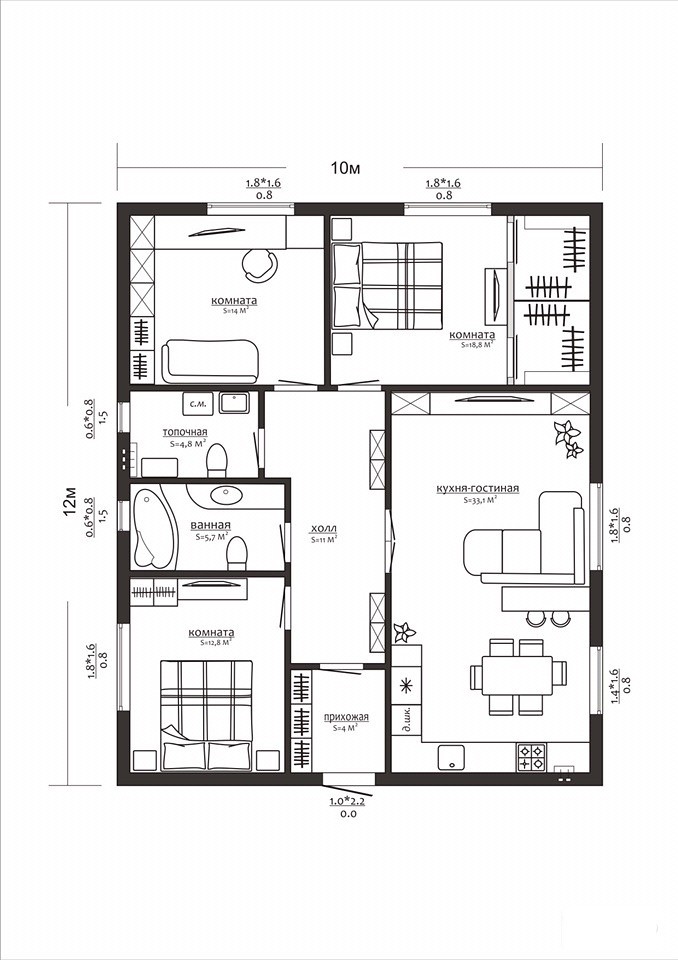This is a detailed blueprint of a residential house, meticulously annotated in Cyrillic script, indicative of Russian architectural design. While the text is not translated, one can discern various rooms and spaces typical of a home layout. The blueprint reveals distinct areas such as a bathroom, living room, bedroom, and a hallway, among others. The detailed floor plan offers a comprehensive view of each section of the house, showcasing the thoughtful design and organization within Russian architectural standards.